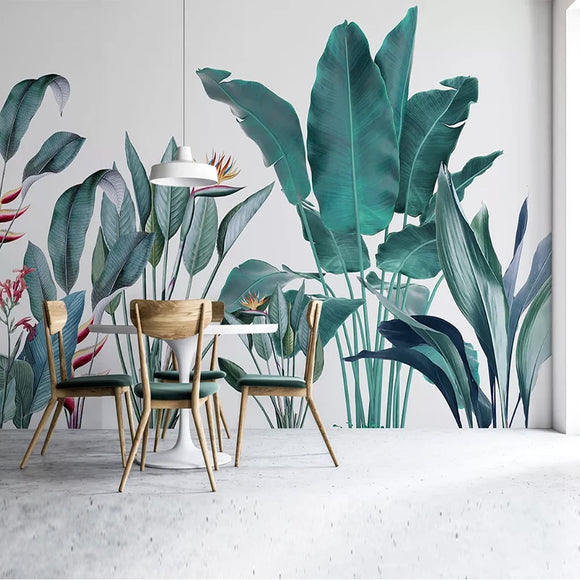The image features a stylish mid-century modern dining room set against an ornate backdrop. Central to the scene is a tulip-style white round table supported by a single pedestal leg, giving it a sleek and minimalist look. Surrounding the table are four wooden chairs crafted from light-colored wood, each adorned with dark green cushions for added comfort. The chair legs splay outward, offering an intriguing design element.

Suspended from the ceiling above the table is a modern, round white light fixture that hangs down on a single cord, providing a soft, even illumination to the room. The floor is a clean, crisp white, enhancing the overall brightness of the space.

Dominating the background is a striking mural on a blue wall, depicting various large tropical plants. Among the plants are vivid illustrations of a bird of paradise, different types of palms, and possibly lilies, characterized by large leaves and vibrant flowers. The mural spans the entire height of the wall, reaching nearly eight to nine feet, creating a lush and immersive natural ambiance within the room.